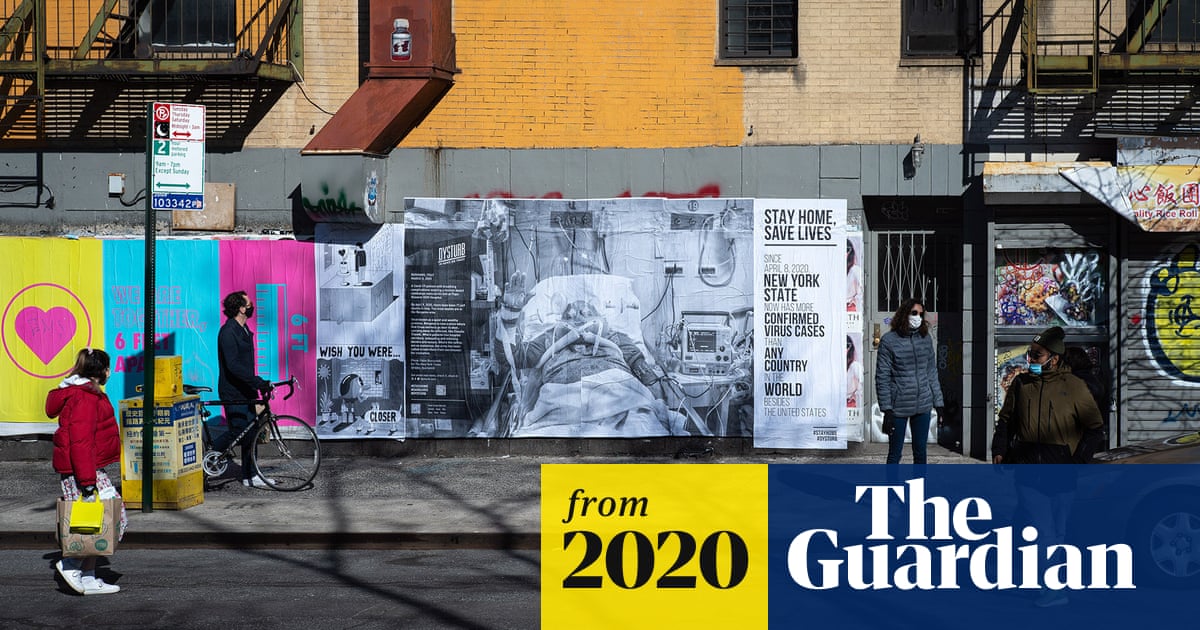The image, sourced from The Guardian in 2020, features a street scene in New York City during the COVID-19 pandemic. On the right side, a woman wearing a blue parka, black slacks, and a face mask stands in front of a door. On the left, a man on a bicycle and a woman wearing a red parka and white sneakers, carrying packages in her right hand, are positioned on the street. They all wear masks, reflecting the period's public health measures. The wall behind them is plastered with posters that include messages like "Stay Home, Save Lives, New York State," and there are also images depicting hospital scenes, emphasizing the gravity of the situation. The bottom right of the image bears the text "The Guardian" in white letters on a blue background and a yellow box with "2020" indicating the year. The scene is completed with visible windows and graffiti, characteristic elements of the urban environment.